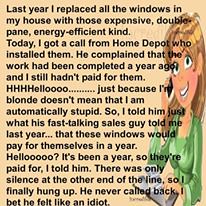The image is a comedic meme featuring a cartoon woman on the right side of a small, tan-colored square. The woman, a brown-haired, smiling white female, is depicted talking on a black mobile phone and possibly typing on a tablet in her lap, dressed in a green blouse. Black text, densely printed across the tan background, tells a humorous story: "Last year I replaced all the windows in my house with those expensive double-pane energy-efficient kind. Today, I got a call from Home Depot who installed them. He complained that the work had been completed a year ago and I still hadn't paid for them. Hello? Just because I'm blonde doesn't mean I'm automatically stupid. So I told him just what his fast-talking sales guy told me last year—that these windows would pay for themselves in a year. Hello? It's been a year, so they've paid for themselves, I told him. There was only silence at the other end of the line, so I finally hung up. He never called back. I bet he felt like an idiot."